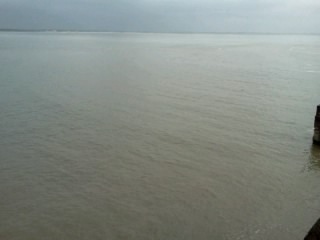The image depicts a vast expanse of calm, dark blue water likely suggesting a sea or ocean, although the stillness of the water could imply a large lake. The water is almost flat calm, with faint, gentle ripples slightly disturbing the surface. The horizon stretches far into the distance, melding seamlessly into a dark blue sky that occupies the top portion of the image, almost blending with the color of the sea. On the right side of the image, particularly in the bottom right corner and near the center, two dark objects, presumably rocks, jut out, hinting at a possible coast. The bottom right corner of the water appears whiter, possibly indicating sunlight shining from above. A thin, dark gray stretch of land or an island can be faintly seen along the far left horizon, adding a subtle geographical reference to the otherwise featureless water.